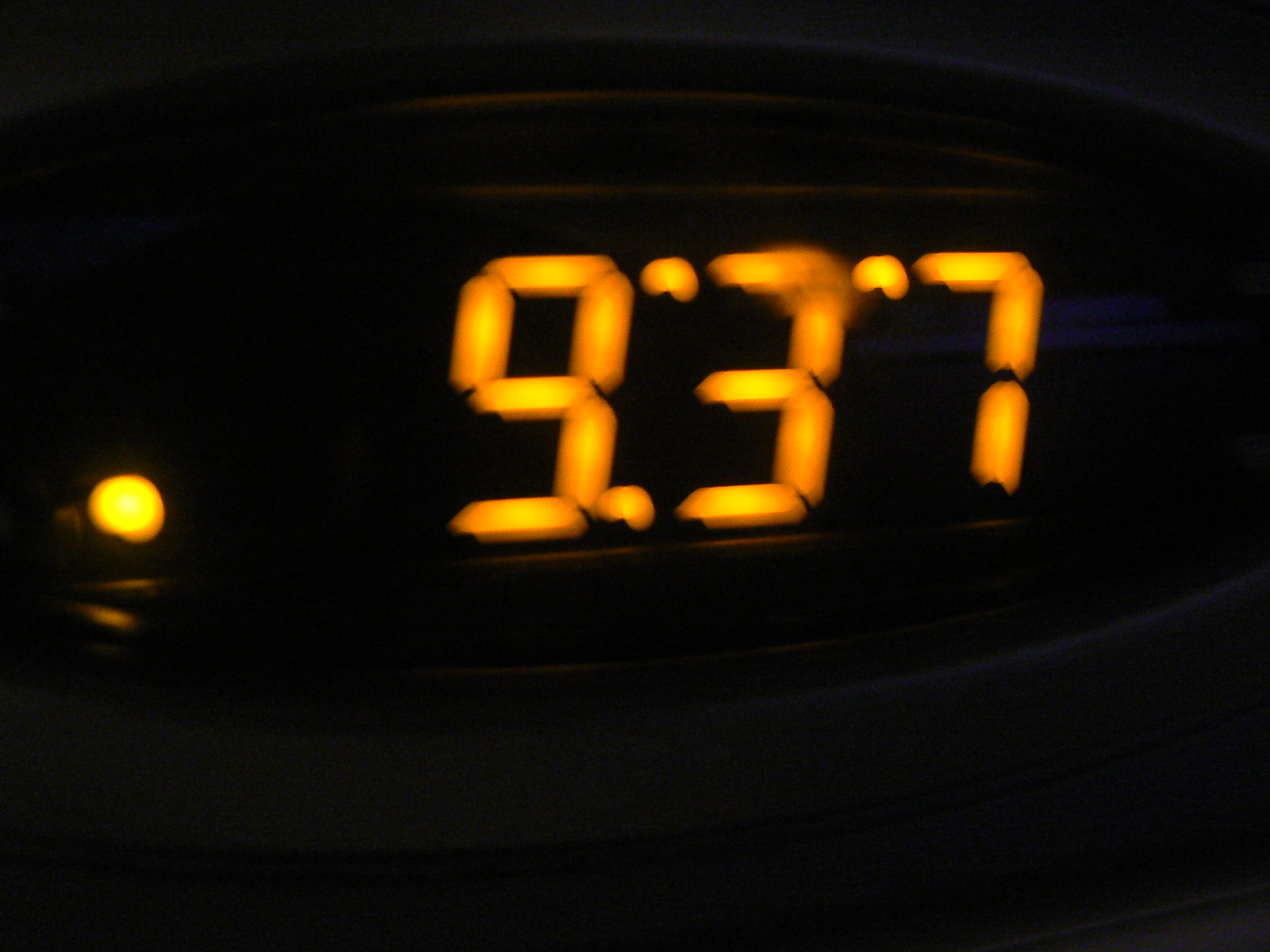This is a very close-up photograph of a red LED digital alarm clock, likely a common household item, displaying the time 9:37. It's a blurry image, making the individual numbers, particularly the "3" and the "7," appear smudged. The clock has a dark black backdrop with a slight bluish shine and is surrounded by what seems to be a silver-colored oval frame, although the low lighting makes this detail hard to confirm. The screen occupies most of the image, showing bright orange glowing numbers. In the bottom left-hand corner, there's a small illuminated dot, probably indicating that an alarm is set. The tight shot and dark lighting obscure additional distinguishing features and any surrounding context.